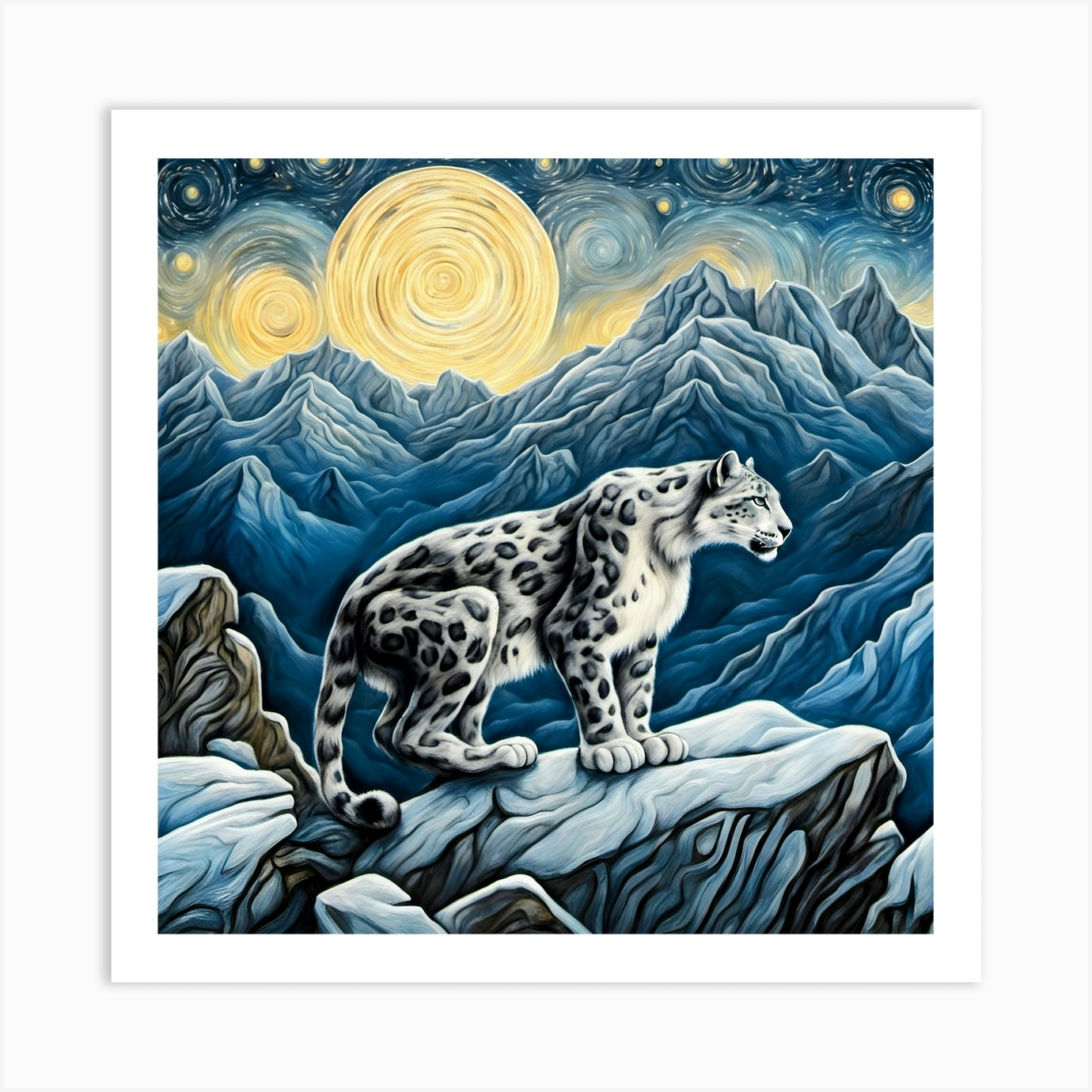This detailed painting depicts a majestic snow leopard, with a grayish-white coat adorned with black spots, poised elegantly atop a snowy rock cliff. The environment merges elements of realism and abstraction, capturing the essence of a snowy, rocky landscape. Beyond the leopard, a series of sharp, icy blue mountains stretch toward the horizon, creating a striking contrast with the richly textured foreground. The sky is a mesmerizing tapestry of circular, sun-like yellow swirls, evoking a sense reminiscent of Van Gogh's Starry Night, and infusing the scene with vibrant movement. The dominant hues of blue, yellow, navy, and light blue blend harmoniously, enhancing the overall dreamlike quality of the artwork, while the leopard gazes confidently towards the right, its long tail trailing gracefully to the left.